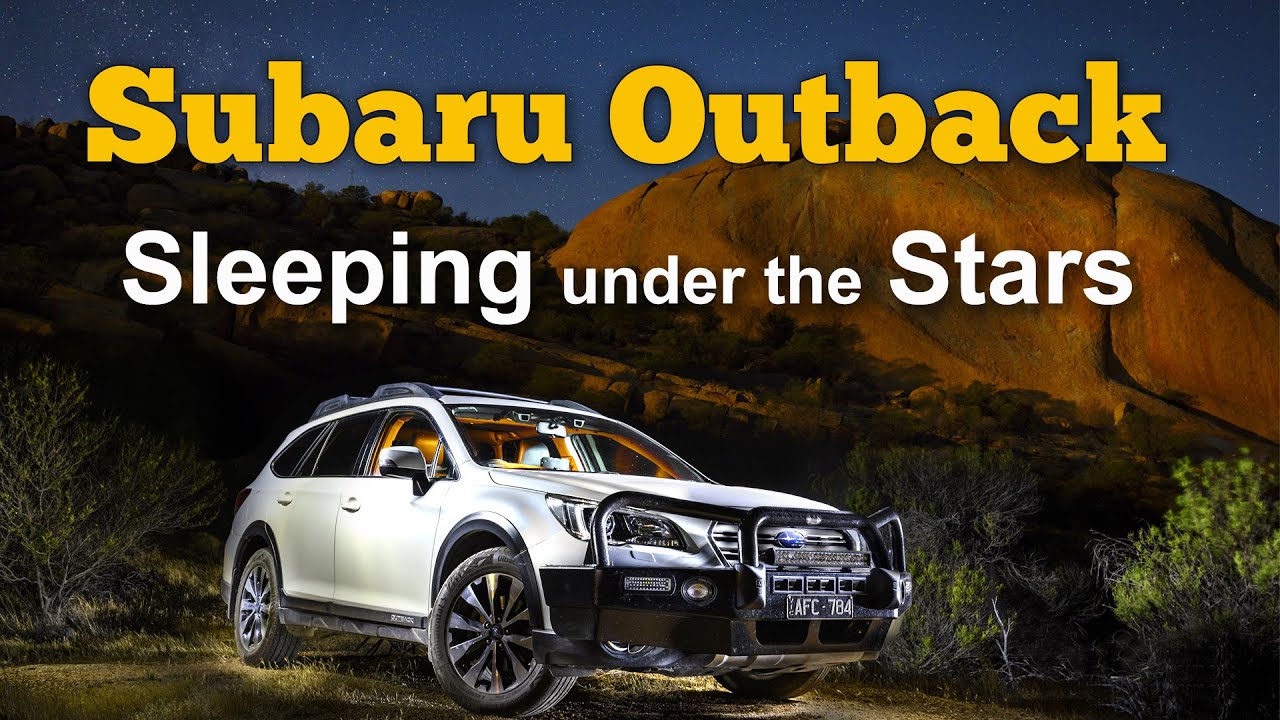In this nighttime outdoor advertisement, the photograph showcases a white four-door Subaru Outback hatchback, positioned prominently on a dirt road at the base of a steep hill. The vehicle, featuring a distinctive black push bar or bumper, is illuminated under a starry midnight blue sky, creating a striking contrast with the surrounding darkness. Green sagebrush frames the scene, stretching across the hill from left to right, adding a touch of wild desert vegetation. A large, red-toned rock formation reminiscent of Uluru in Australia dominates the upper right portion of the image. Large yellow text at the top of the graphic reads "Subaru Outback," with the tagline "Sleeping Under the Stars" in bold white print just below, capturing the adventurous and rugged spirit of the vehicle. The entire banner, roughly five inches wide by three inches high, encapsulates the essence of an off-road escapade, inviting viewers to embrace the thrill of nighttime exploration.